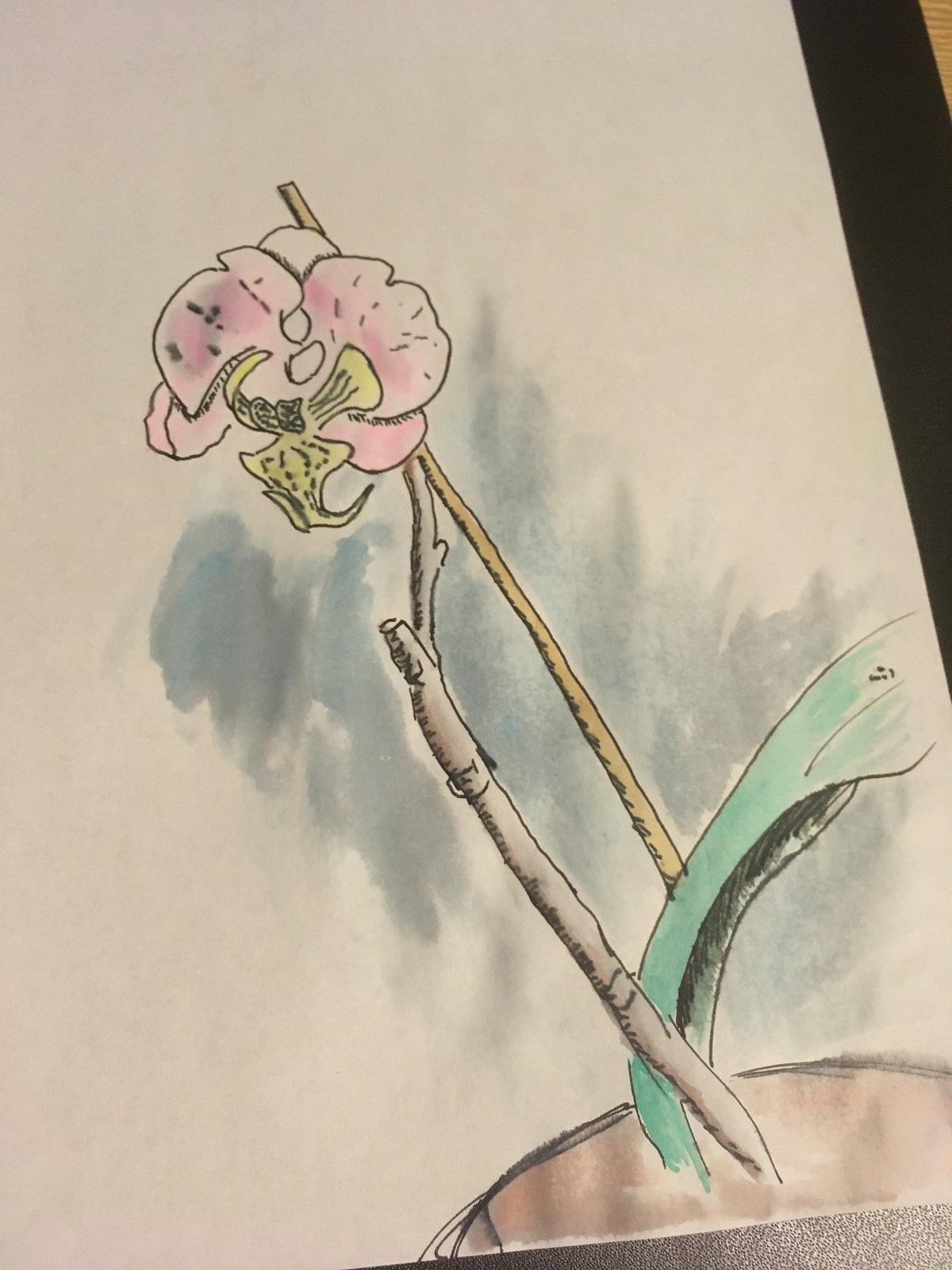This photograph captures a beautifully detailed piece of artwork that features a flower, possibly an orchid or lily, rendered in a combination of dark pencil or pen outlines and watercolor paints. The flower, delicately positioned in the bottom right corner of a pristine white sheet of paper, emerges from a modest brown mound of dirt. Ascending from this mound is a slender brown stick, accompanied by a vibrant green leaf and a light tan stick that lends support to the flower's stem. The blossom itself showcases light pink petals with a soft yellow center, while subtle blue and gray brushstrokes suggest a serene sky in the background. The artist's meticulous attention to detail and skillful use of color bring the flower to life, creating a tranquil and enchanting scene.